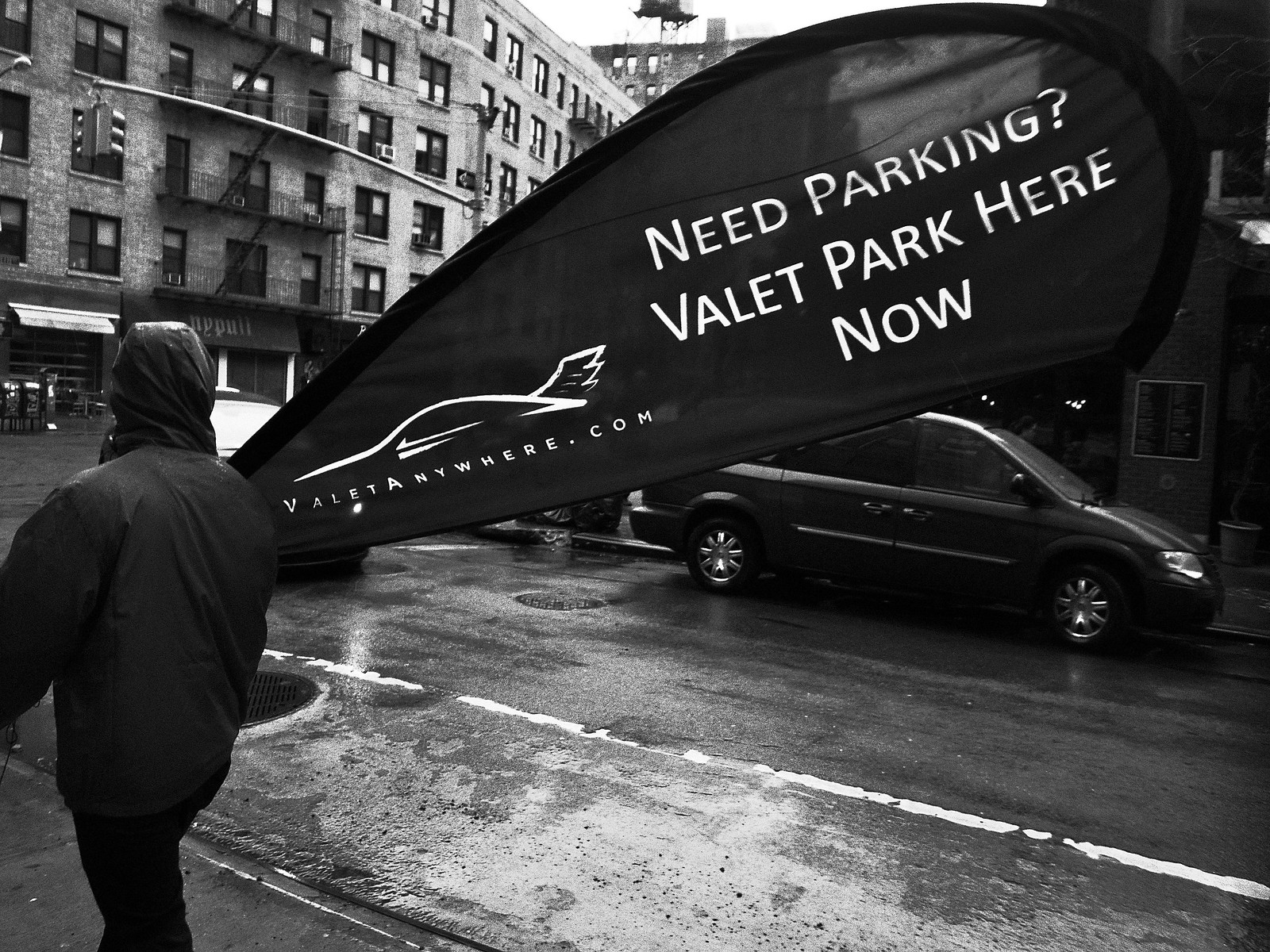This black and white photograph captures a gray, overcast, and potentially rainy day in the city. In the foreground, a man is walking down a wet street, dressed in a dark raincoat with the hood up, concealing his face. The dominant feature he carries is a large, dark-colored sign that reads "Need parking? Valet Park here now" in white text, alongside the logo and URL "valetanywhere.com." A multi-story stone building with connected shopfronts serves as the backdrop, adding urban character to the scene. Additionally, an SUV with silver-spoked wheels is noticeable parked or moving slowly behind the man, complementing the dreary urban landscape.